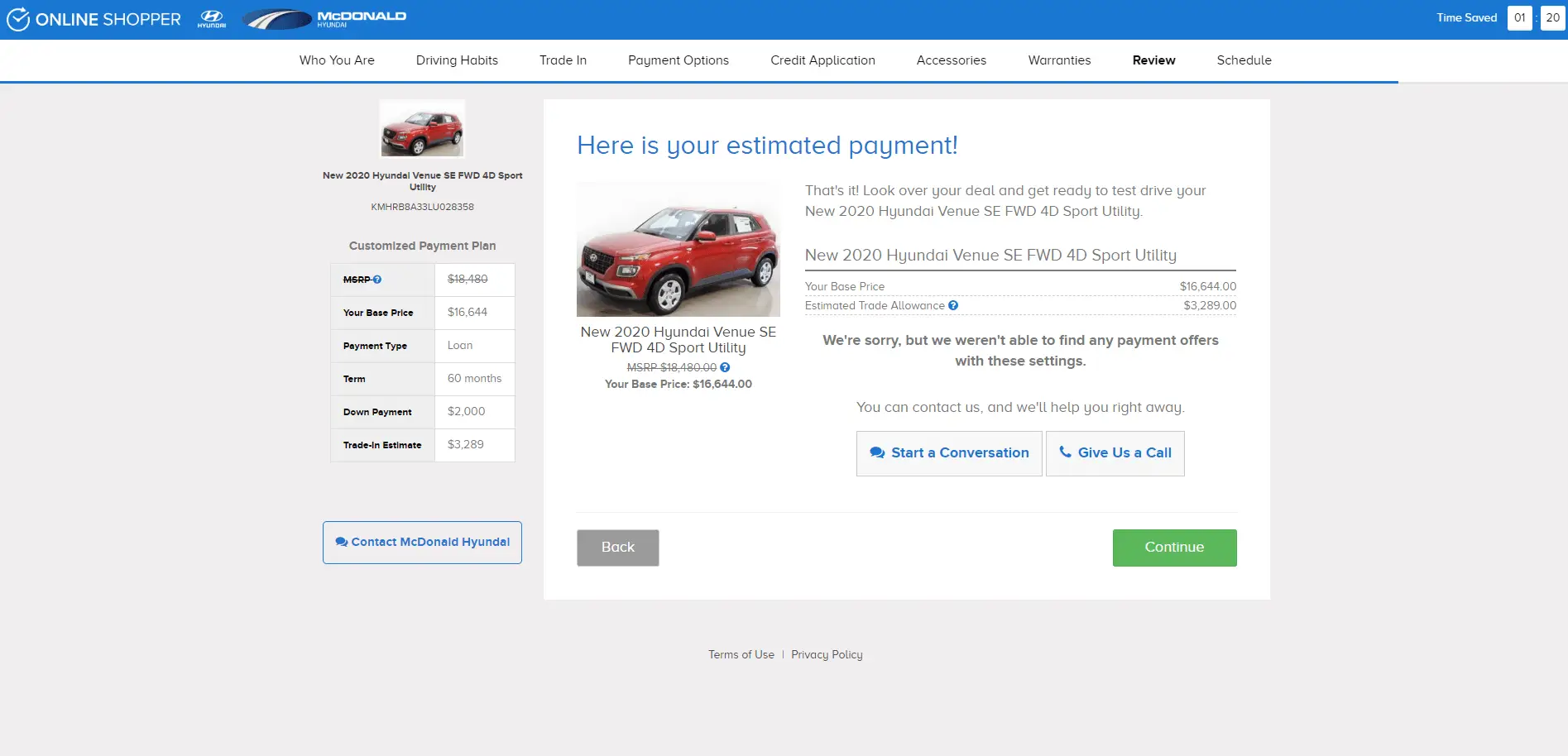This image appears to be a screenshot from a website designed for online car shopping, specifically on a phone interface. The entire page has a predominately light gray color scheme. At the top, there is a narrow dark blue border approximately half an inch in height, followed by a similar width white border beneath it. Within the dark blue section, a white circle is visible, containing a check mark in the top right corner of the circle. Adjacent to this, in white text, are the words "Online Shopper."

Below this, the Honda emblem is featured prominently, accompanied by the brand name "Honda." Positioned further down, another blue circle showcases a stylized road stretching diagonally from the lower left to the upper right within it. To the right of this circle, "McDonald" is written in bold white letters, while underneath in smaller text, "Hyundai" is displayed.

On the left side of the page, the words "Time Savings" are rendered in white. Further down, a white square contains the numbers "0-1," followed by another white square with the numbers "2-0" in black. Along the blue border stretching across the white background, nine drop-down tabs can be seen, with labels such as "Who You Are," "Driving Habits," "Trade-in," etc.

Under the "Driving Habits" tab, a small picture of a white car facing left is visible, including details about the vehicle's cost, miles per gallon, and other specifications. At the bottom of this section, a light gray tab with a blue border states "Contact McDonnell Hyundai," while to its right, a white square is labeled "Your Estimated Payment!" in the top blue left corner, followed by another image of the car also facing left, presenting further details about the vehicle's price and type.

To the left of this section, information is provided regarding test-driving the car, its cost, estimated allowance, and additional offers that may not be available at the moment. Lastly, at the bottom, a gray tab with blue lettering prompts viewers to "Start a Conversation," situated beside another gray tab encouraging them to "Give Us a Call." In the bottom left corner, a black tab with "Back" written in white is present, and on the right, a green tab with "Continue" printed in white concludes the interface layout.